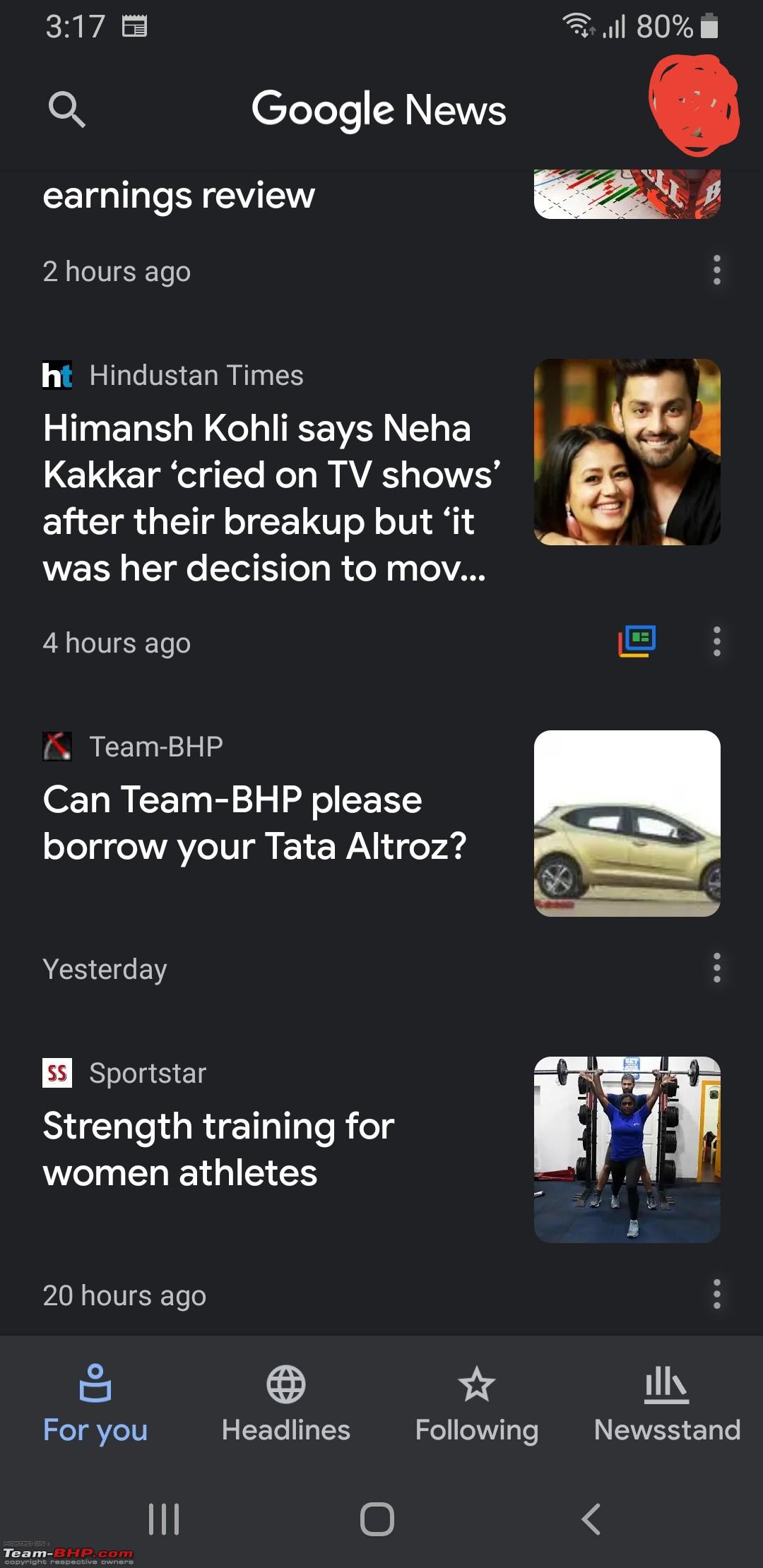A screenshot from Google News on a mobile device displays various features and articles. At the top center of the screen, the Google News logo is prominent, flanked by a search button on the left and a user profile icon on the right, which has been obscured with a red digital scribble. Below the logo, several news articles are listed. The top article is partially visible, concluding with the phrase "earnings review from two hours ago." The next article, from the Hindustan Times, is titled "Himansh Kohli says Neha Kakkar cried on TV shows after their breakup when it was her decision to move," posted four hours ago. Following this, an article from Team BHP appears with the headline "Can Team BHP please borrow your Tata Altroz?" posted yesterday. The final article, from Sportstar, is titled "Strength Training for Women Athletes," posted 20 hours ago.

At the bottom of the screen, four navigation buttons are displayed: "For You," "Headlines," "Following," and "Newsstand." Below these, three additional buttons are positioned: a menu represented by three horizontal lines on the left, a home button in the center, and a back arrow on the right.